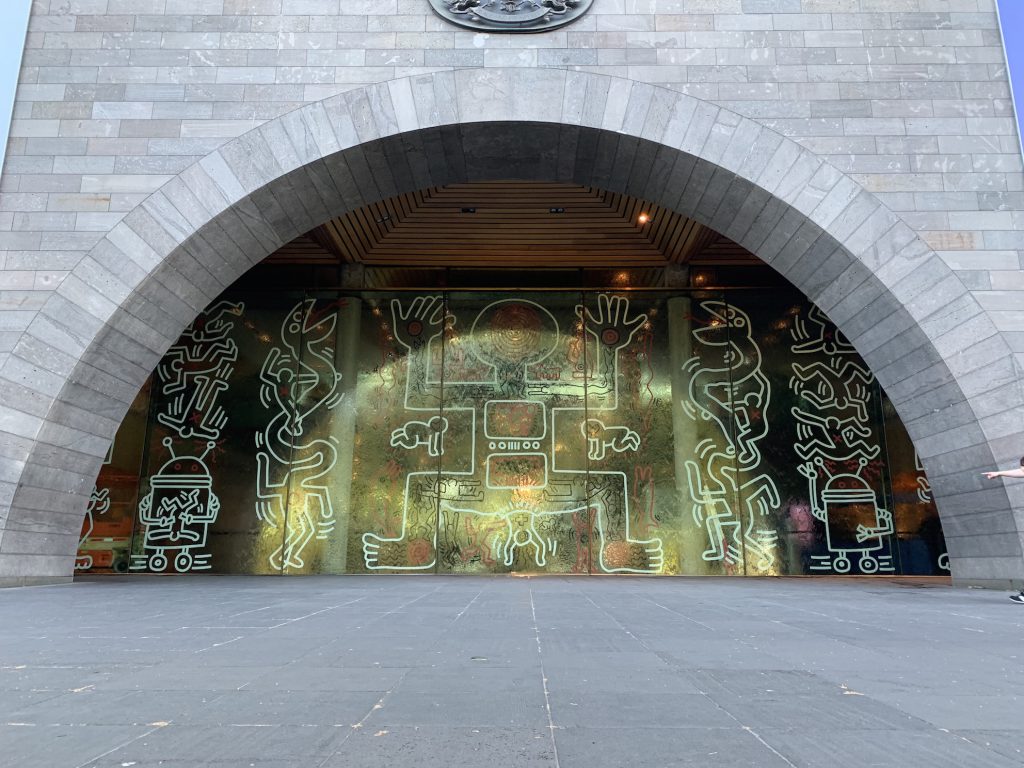The photograph, taken at a low, almost ground-level angle, captures an intricate scene dominated by a stone building with a prominent archway. The ground is covered with grey square paving stones, irregularly colored and littered with dirt and detritus, while subtle pink elements peek from where grout might be. The archway of the building features an array of multi-colored bricks—shades of grey, beige, rustic tones, and light blues. Just above the arch, a small sliver of a metallic emblem is visible, though partially cut off by the frame. Directly beneath the arch, the face of the building showcases glass panels adorned with white, Keith Haring-inspired doodles. The central figure of the artwork is a man with arms and legs splayed, surrounded by peculiar illustrations including aliens, robots, snake heads, and figures crawling out from him, evoking a sense of surrealism. The panels above the artwork and between the arch reveal square slats with spotlights, creating reflective patterns on the glass. To the right side of the image, an arm extends into the frame, pointing towards the central drawings, adding an element of human interaction to the scene. While part of a circular shape is visible at the very top, the intriguing composition of the image remains cut off, adding to its enigmatic allure.